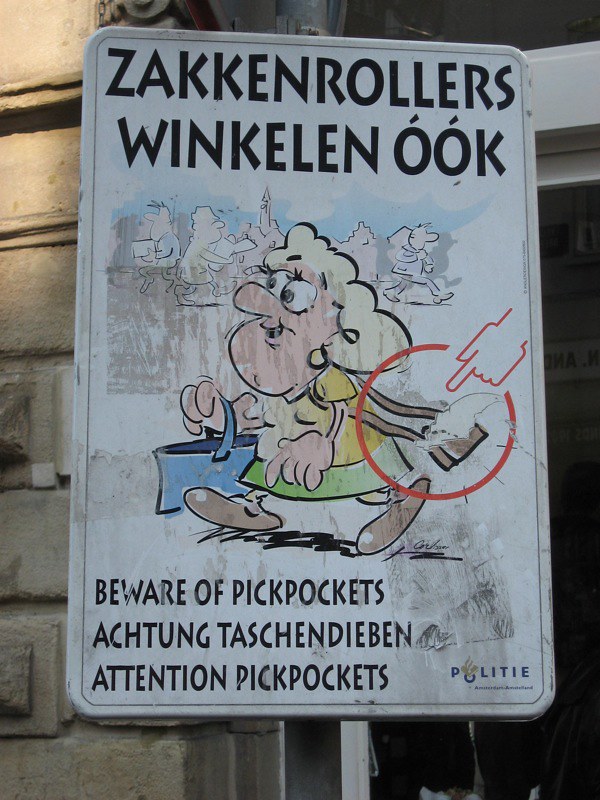The image is a photograph taken outdoors, capturing an old, worn warning sign with chipped paint. The sign is white and mounted on a light brown post, with bold black capital letters at the top reading "Sack and Rollers will win killin ook." The sign also features a cartoon illustration of a blonde woman in a yellow shirt walking, holding a blue bag with her purse loosely dangling behind her. A hand is pointed at her purse, emphasizing the warning message about pickpockets. In the bottom left corner, the text reads "Beware of pickpockets Achtung Daschendieben Attention pickpockets." The bottom right corner includes a phrase in another language, possibly "a politay."